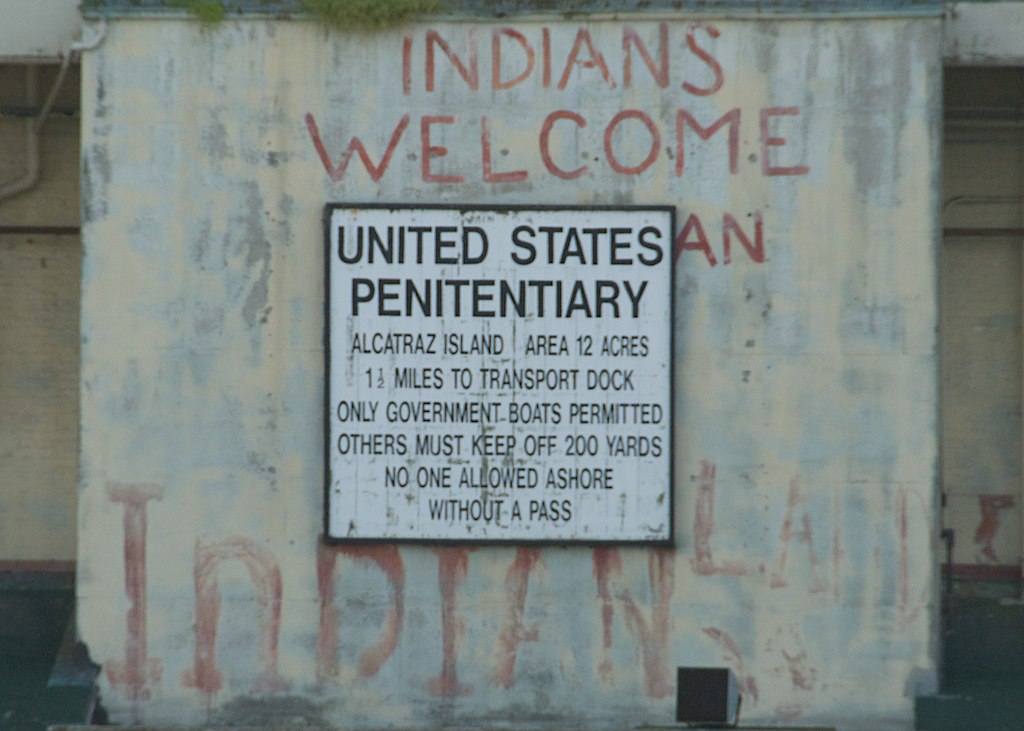This is a full-color outdoor photograph of a dilapidated concrete wall, possibly part of an abandoned building. Dominating the center of the image is a white sign with a black border, containing black text that reads: "United States Penitentiary. Alcatraz Island, area 12 acres, 1.5 miles to transport dock. Only government boats permitted. Others must keep off 200 yards. No one allowed ashore without a pass." Above this sign, hand-painted in red, is the phrase "Indians Welcome." Towards the bottom, also hand-painted in a faded and sloppy script, is the word "Indian." The concrete wall appears weathered, with a brownish structure visible on either side and a pipe protruding from the left. The overall color palette includes tones of gray, white, black, red, and beige, contributing to the image's aged and rugged aesthetic.